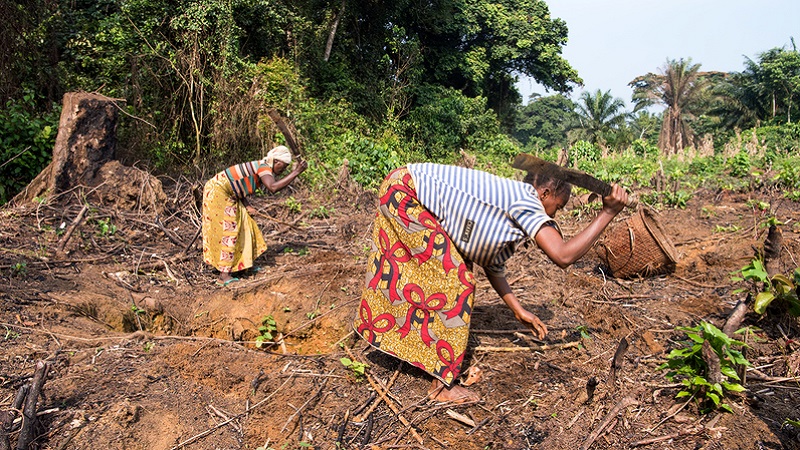In this bright, sunny outdoor photograph taken at ground level, two black women are captured in a rugged, untamed field. They kneel close to the rough, predominantly dirt ground, which is strewn with numerous twigs and branches, devoid of almost any grass. The women are dressed in vibrant, patterned green dresses, consisting of skirts and short-sleeve shirts. Each woman holds a machete poised behind her shoulder, seemingly ready to strike at the ground. On the right side at the bottom of the image, a section of a cut, thin tree trunk with leaves is visible. Surrounding the scene, there is an array of foliage, including bushes, palm trees, and various other trees, some of which appear to be dead, with the sky peeking through in the upper right corner in a pale, light blue hue. The backdrop suggests an effort to clear or prepare the rough terrain for future use.